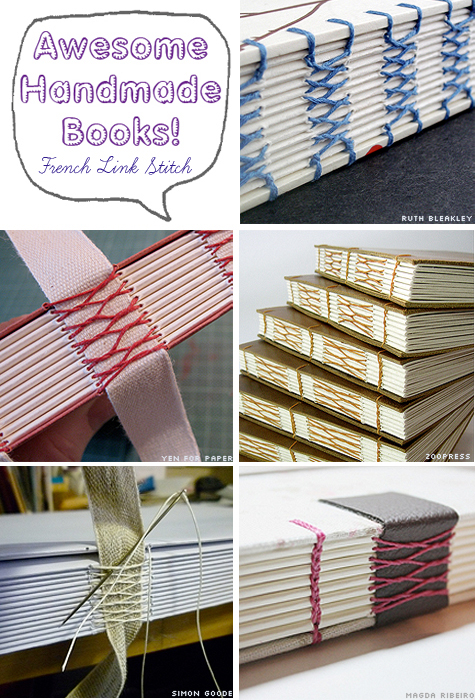The vertically oriented image features a grid of six perfect squares, arranged with two across and three down. In the top-left square, there's a white background with a hand-drawn speech bubble, outlined in black, possibly created using colored pencil or crayon, containing purple text that reads, "Awesome Handmade Books, French Link Stitch." This indicates a guide on making handmade books using the French link stitch method. The remaining five squares showcase various examples of the stitch techniques on handmade books. The second square (top-right) displays a book with royal blue stitching. Directly below it (middle-right square), there is another book with a yellow stitch pattern along its edge. The middle-left square features a book with a red stitch pattern. In the bottom-left square, there is a beige piece of thin fabric with a needle and thread visible through the stitch pattern, resembling a woven belt. The final square (bottom-right) depicts a book with a gray binder adorned by pink threaded stitches. The showcased patterns and colors—blue, red, yellow, pink, white—demonstrate the diversity and creativity of handmade bookbinding using the French link stitch.